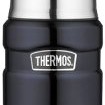This image is a small, possibly computer-generated or screenshot, displaying two thermoses sitting next to each other on a plain white background. Both thermoses have black plastic grips and silver chrome caps. The black plastic grips feature raised lines that run vertically down their centers, possibly indicating three separate black strips. The equally spaced black lines create a symmetrical appearance, with the central line intersecting the "R" and slightly the "M" in the word "THERMOS," prominently displayed across the middle of the thermoses. The thermos logo appears in silver against the black background, positioned between the grips that encircle the thermoses, emphasizing their functional yet sleek design.